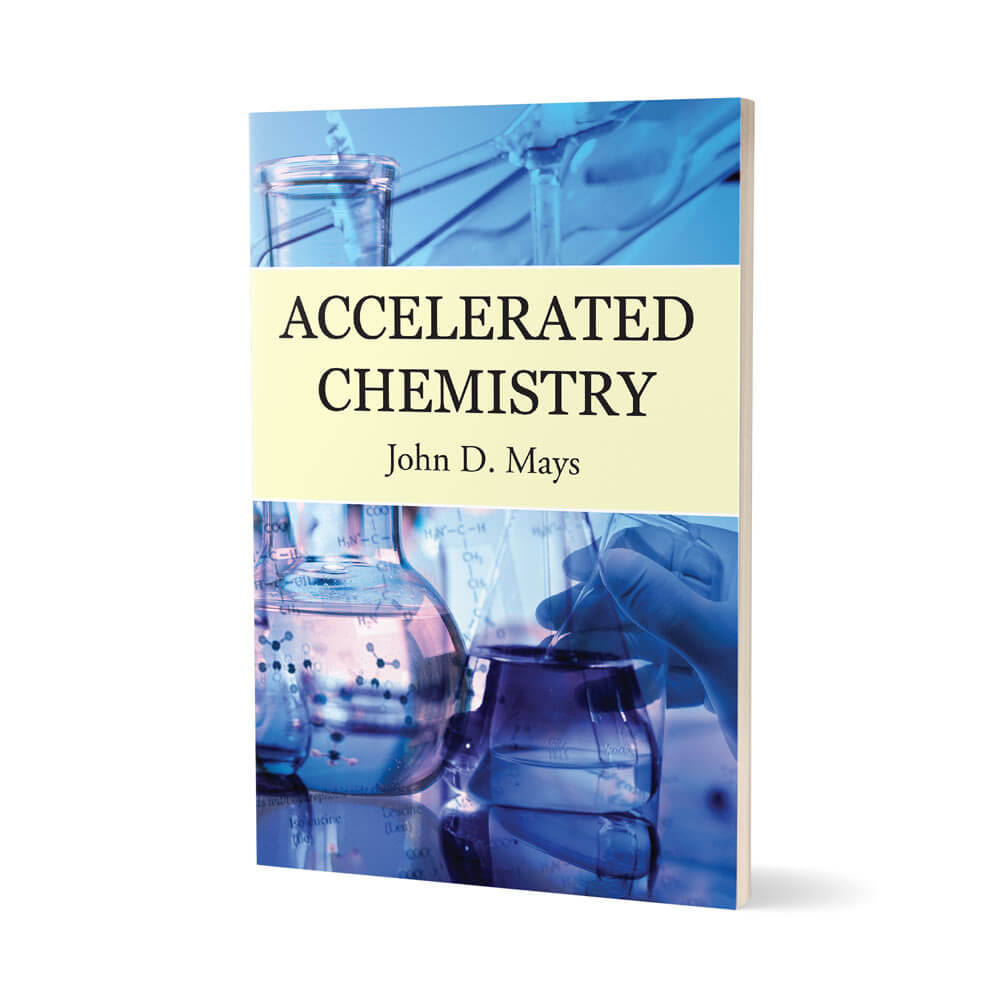The image showcases the front cover of a paperback textbook titled "Accelerated Chemistry" by John D. Mays. The book is positioned upright against a solid white background, giving it a floating appearance within an empty white void—likely indicative of a product display for a sales page. The cover, dominated by a photograph under a pink and blue filter, presents a scene of someone handling various lab beakers filled with clear liquid, suggesting an ongoing experiment. Central to the cover is a horizontally running tan banner with bold, black text that reads "ACCELERATED CHEMISTRY" in all caps, followed by the author's name, "John D. Mays," in smaller font. The photograph also features molecular structures and organic chemistry chains sketched on the beakers, enriching the scientific theme. The background of the image transitions from blue at the top to purple at the bottom, further enhancing the visual appeal. The book appears to be about five inches tall and three inches wide, with the right side angled closer, revealing the pages inside.